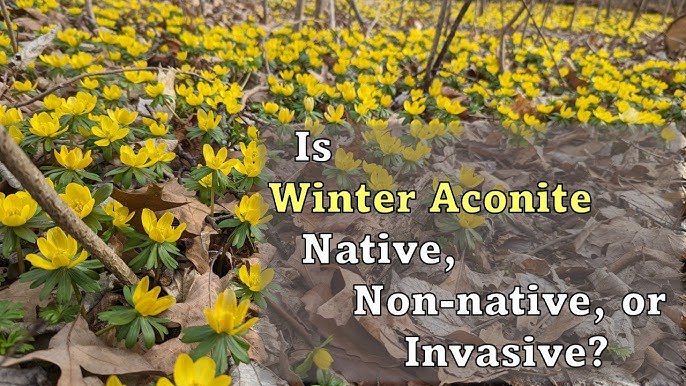The image depicts a dense carpet of cheerful yellow flowers, identified as winter aconite, blanketing what seems to be a forest floor. Each flower features multiple upright petals, surrounded by deep green leaves that closely resemble the petals but extend more horizontally. Interspersed among the vibrant flora are tree saplings and dry, fallen leaves, suggesting an autumnal setting. The forest floor is dotted with brown tree stumps, adding texture and complexity to the scene. In the lower right-hand corner, a watermark questions, "Is winter aconite native, non-native, or invasive?" rendered in large white font, with "winter aconite" standing out in yellow. This text is slightly blurred into the background, hinting at an inquiry possibly prompted by the profusion of blossoms stretching as far as the eye can see.